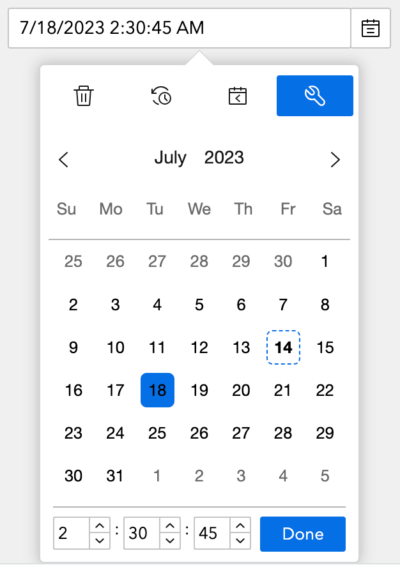The image features a calendar page for July 2023. At the very top of the image, within a white rectangle with black text, the precise date and time are displayed as "07-18-2023, 2:30:45 AM". Below this, in the upper left corner, there are several icons: a trash can, a clock with an arrow indicating a reset or redo function, a calendar, and a wrench within a blue square. The main section of the calendar shows the month "July 2023" prominently. The days of the week—Sunday, Monday, Tuesday, Wednesday, Thursday, Friday, and Saturday—are laid out across the top. The date "July 18th" is highlighted with a blue square featuring rounded edges around the number 18. At the top right of the image, the current time is reiterated, and next to it is a rectangular button labeled "Done".